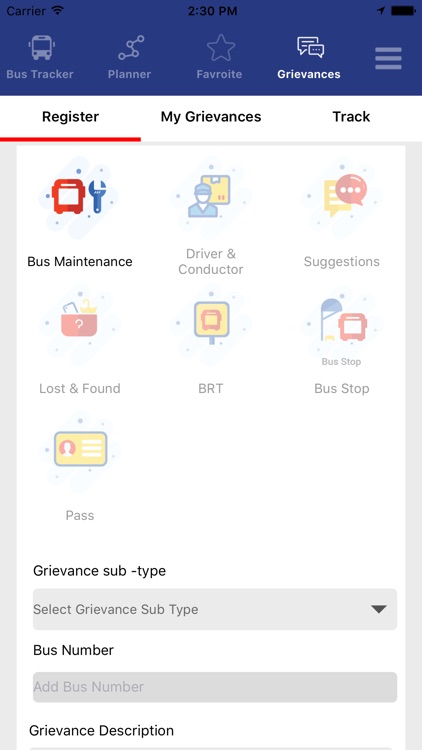This image appears to be a detailed screenshot of a mobile application's interface, possibly a transit app. The screenshot is in portrait orientation, typical of images taken with an iPhone or Android device. 

At the very top of the screen is a large navy blue rectangle containing system status information. In black letters, it reads "Carrier" with a Wi-Fi symbol next to it. Centrally located within this rectangle is the time, "2:30 PM." On the far right side, there's an upward-facing triangle adjacent to a fully charged battery icon.

Directly below this header is a functional area of the app showcasing four actionable icons. The first icon is a gray bus labeled "Bus Tracker," featuring a connected series of circles forming a Z-shape. Below it, another icon labeled "Planner" is visible. Next, a star icon labeled "Favorite," followed by a white-highlighted icon of two speech bubbles with the word "Grievances."

Beneath these icons is a menu with three options: "Register" in black letters highlighted with a red bar below it, "My Grievances" in black letters, and "Track" on the far right.

In the middle, there is a large white area predominantly labeled "Bus Maintenance" featuring a red bus icon next to a blue wrench on a gray background. The adjacent icons are grayed out. To the right of "Bus Maintenance," there is an icon of a person in a uniform with a yellow square above their right shoulder, marked "Driver" and "Conductor" in gray letters. Further to the right, an icon combining a yellow text bubble with white bars and a red speech bubble with three white dots is labeled "Suggestions."

The next row contains three items: a red bin with a question mark and some items protruding, marked "Lost and Found" in gray letters; a yellow-background icon with a red bus surrounded by a blue outline labeled "BRT" in large black letters; and a "Bus Stop" icon featuring a blue lamppost with a red bus next to it, labeled the same in smaller letters above.

Towards the bottom of the screen, on the lower-left corner, an icon labeled "Pass" with a yellow rectangle outlined in blue and a white person icon against a red background with three white bars. Below this, in black letters, is "Grievance Subtype" next to a long gray bar for selection. The gray text inside reads "Select Grievance Subtype," accompanied by a downward-pointing triangle. Below this section, the words "Bus Number" precede another long gray bar with faint gray letters reading "Add Bus Number."

The bottommost section starts with "Grievance Description" in black letters, which gets partially cut off. The entire interface is outlined in gray on both left and right sides.